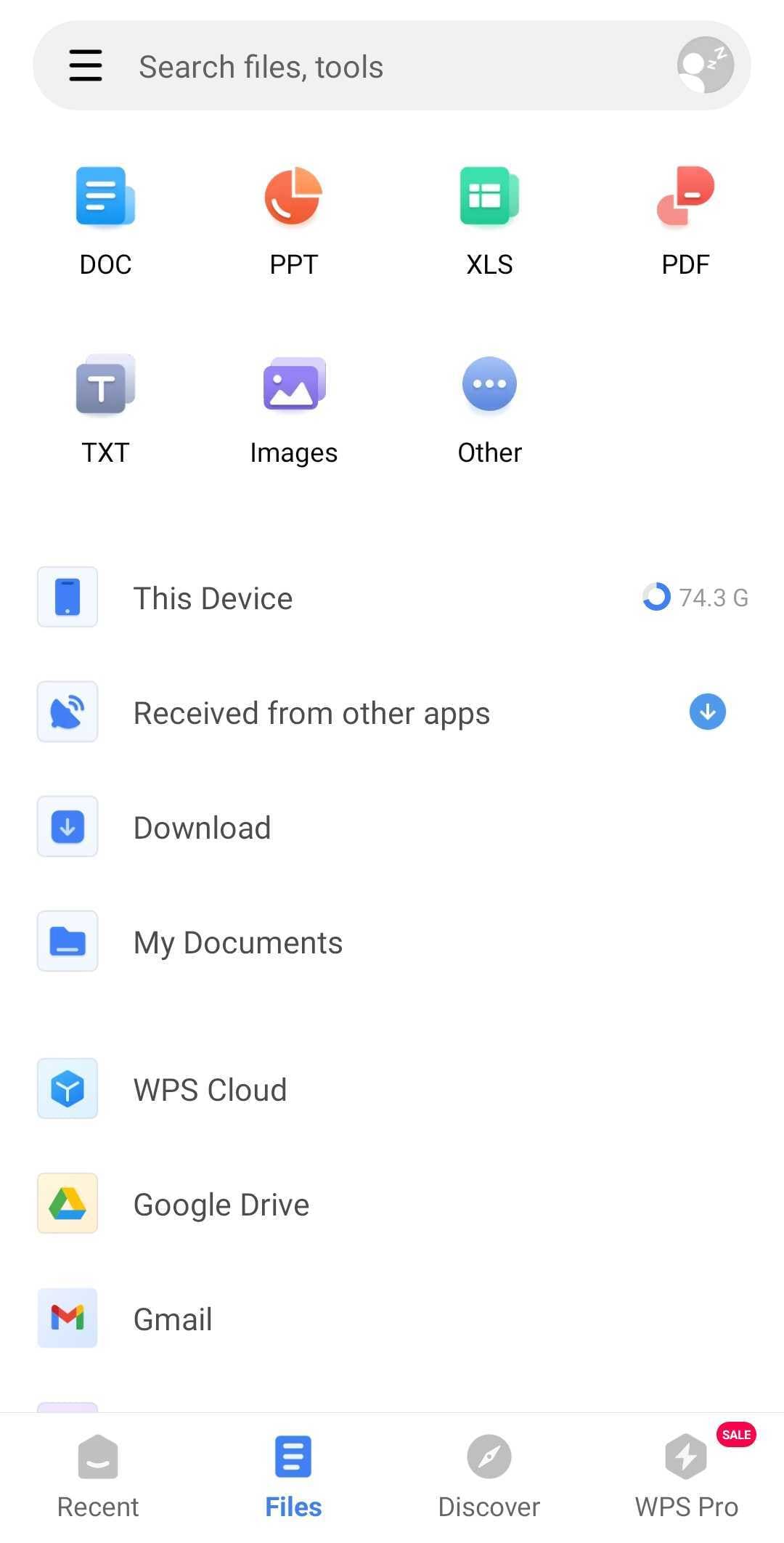In this image, there is a prominent white background. At the top of the image, a blue rectangular box contains three black horizontal lines alongside the text "Search files and tools." Adjacent to this text, there is a small circular icon featuring a person's silhouette.

On the main white background, several file format icons are displayed: DOC, PPT, XLS, PDF, TEXT, IMAGES, and OTHER. Below these icons, a device is depicted with a storage display showing "74.3 GB." A circular progress indicator is approximately two-thirds filled with blue.

Further down, there is a section labeled "Received from other apps," marked by a blue circle with a downward arrow inside it. Additional options include "Download," "My Documents," "WPS Cloud," "Google Drive," and "Gmail." 

At the bottom of the image, there is a navigation bar with four options: "Recent," "Files," "Discover," and "WPS Pro." A small pink box is situated above this navigation bar.